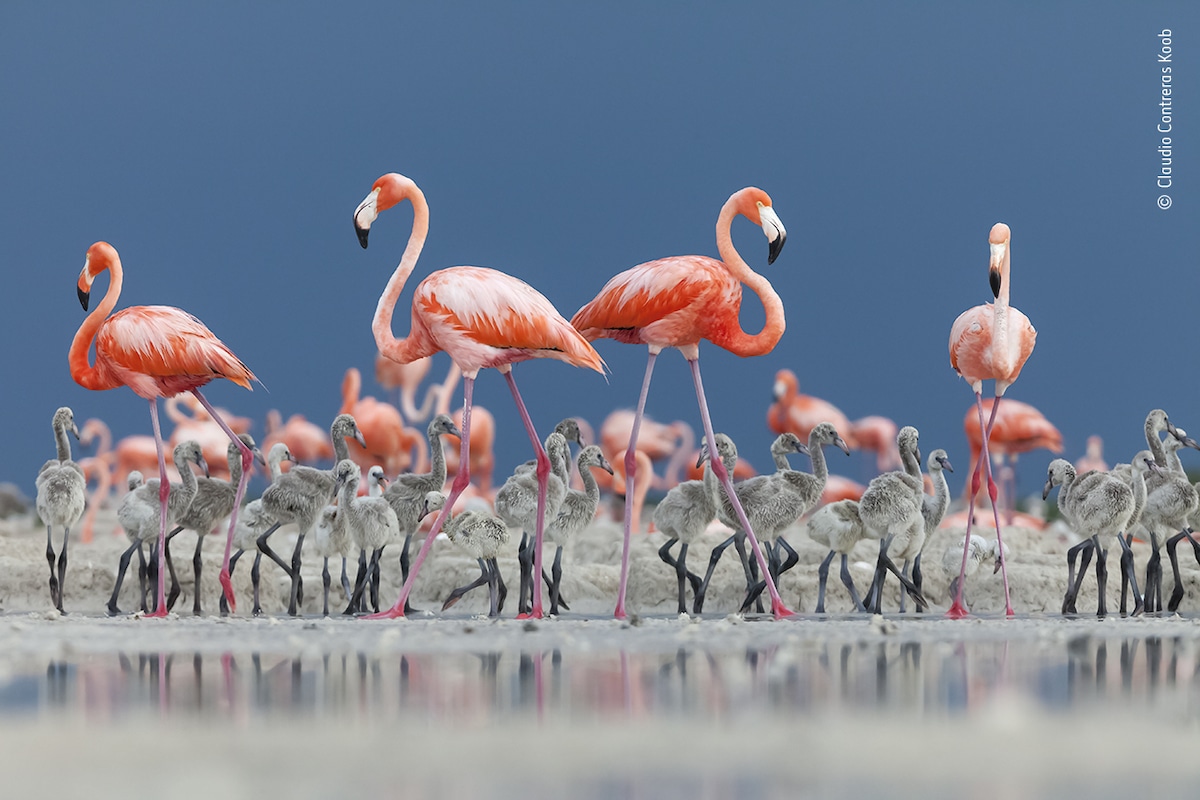This is a professional photograph by Claudio Contreras-Koob, showcasing a stunning scene of flamingos and their chicks. In the foreground, a blurred surface of water gives way to a gray sand beach where four vibrant pink adult flamingos stand elegantly, surrounded by a couple dozen gray flamingo chicks with thin black legs. The flamingos' tall, skinny legs appear purplish with pink joints, leading up to their round, coral-colored bodies adorned with rich pink feathers and white accents. The adult flamingos have long, curved white beaks tipped with black. The background is a blurred slate blue sky, and additional flamingos can be seen, slightly out of focus. Reflections in the water and the slight upward perspective create a sense of depth, making the viewer almost level with the birds. The photograph captures the tranquil yet lively interaction between the adult flamingos and their adorable, gray-feathered chicks, standing poised at the edge of the water—a striking composition of nature’s beauty. In the top right-hand corner, the copyright notice of Claude Contreras-Ku is visible, asserting the photographer's credit for this beautiful image.